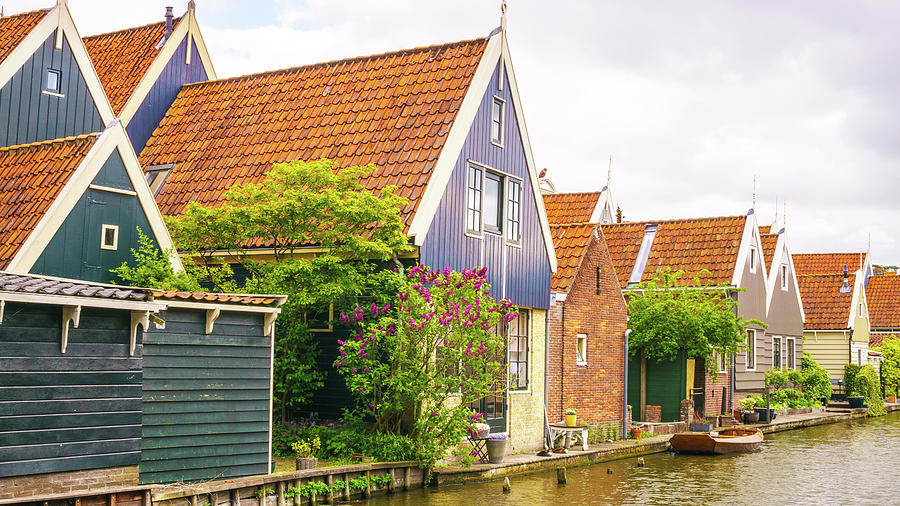The image depicts a charming row of houses or cottages lined up directly beside a waterway, creating a picturesque village scene. Each house has a square base and a triangular roof, resembling a tall A-frame structure, with roofs uniformly covered in brown shingles. The exteriors of these homes vary in materials and colors, including wood and brick, with hues of blue, yellow, beige, and traditional brick red. Between the houses, lush greenery, including trees and flowering bushes with pink blossoms, adds a vibrant touch to the scene. Nestled on the walkway behind the houses is a small brown rowboat or canoe, capable of seating two to four people, emphasizing the quaint riverside setting. The waterway itself runs brown and muddy right up to the greenery, and the sky above is filled with white, puffy clouds in various shades of white, blue, and gray. There are also outdoor tables and chairs arranged beside some of the houses, enhancing the cozy and inviting atmosphere of this tranquil village. No people are visible in the image, focusing the attention solely on the charming architecture and natural beauty of the setting.